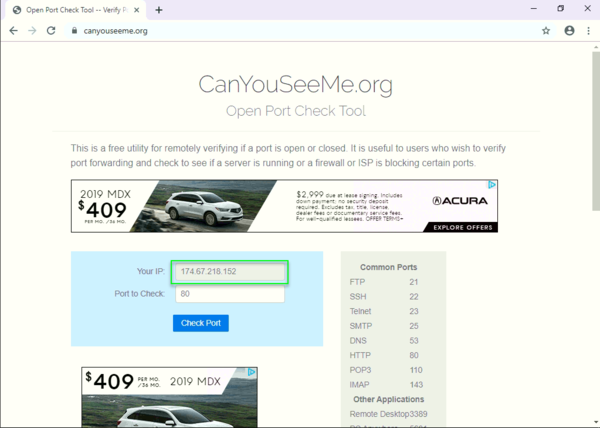The image depicts a screenshot of the website "canyouseeme.org," which is housed within the URL button at the top of the screen. To the left of this URL button, there is a sequence of navigation and security icons including a left arrow, a right arrow, a refresh button, and a lock symbol. Further to the right are a star icon, a user icon, and a menu icon with three vertical dots.

Dominating the main section of the page, "canyouseeme.org" is displayed prominently in large, bold letters on a white background. Below this, in slightly smaller text, it reads "Open Port Check Tool." The description beneath explains that this is a free utility designed to remotely verify if a port is open or closed, which is particularly valuable for users wishing to verify port forwarding, check server operations, or determine if a firewall or Internet Service Provider (ISP) is blocking certain ports.

In the middle of the page, there is an advertisement showcasing a 2019 Acura MDX SUV, available for $409 per month. The ad includes an image of a white Acura SUV and a clickable link saying "Explore Acura Offers," allowing users to view more details.

Further down, a blue box displays the user's IP address, with a white rectangular area highlighted in green showing "174.67.218.152." Below this, the text "Port to Check: 80" appears in a separate row, followed by another blue box labeled "Check Port."

Adjacent to these elements, a gray area titled "Common Ports" lists various port numbers and their features within a vertical grayish box. A smaller version of the Acura advertisement is located in the lower left corner of the page.